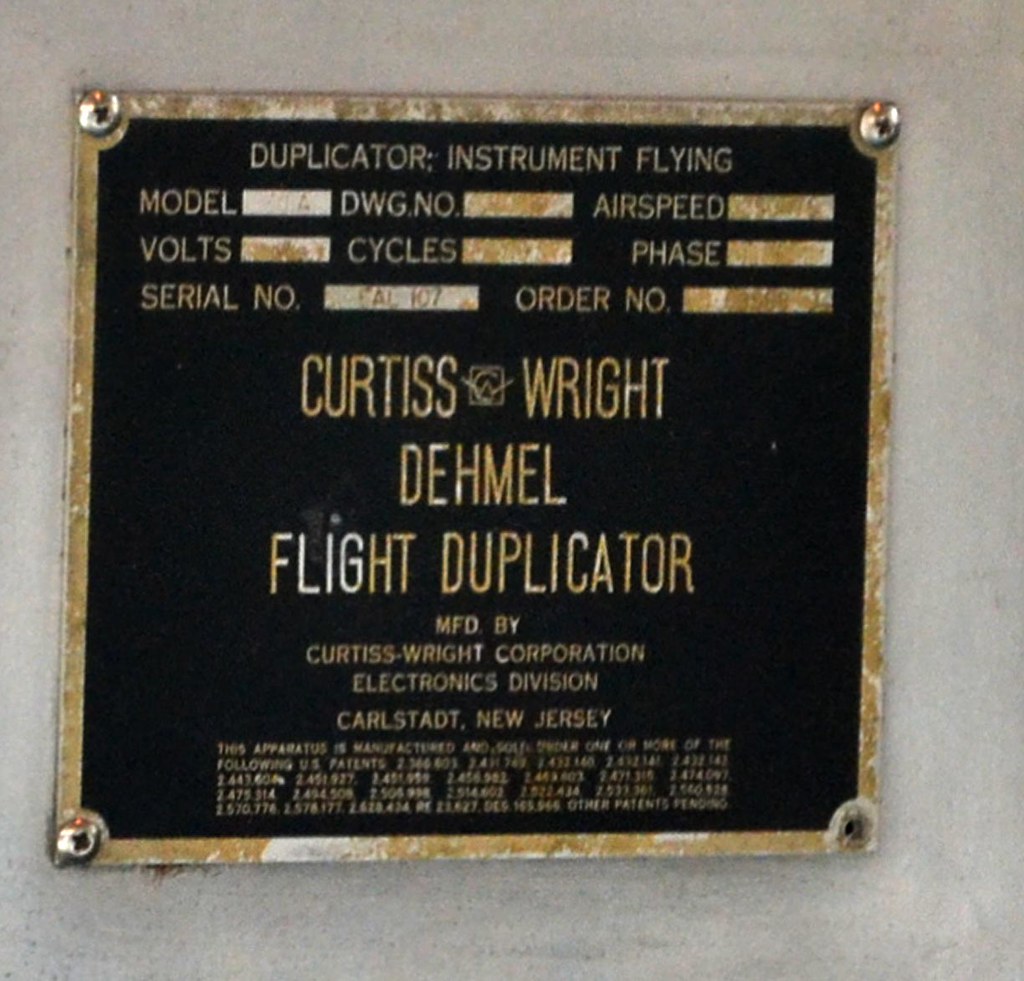This close-up image captures a sleek plaque mounted on a white wall with four silver screws. The plaque boasts a black background framed in gold, featuring elegant gold text. At the top, it reads: "Duplicator Instrument Flying Model DWG.NO, Airspeed, Volts, Cycles, Phase, Serial Number, and Order Number." Below, in larger letters, it states "Curtis Wright Demel Flight Duplicator" and beneath that, "MFD by Curtis Wright Corporation Electronics Division, Carlstadt, New Jersey." The bottom section contains a paragraph in very small, unreadable print, adding further detail to this meticulously designed plaque.